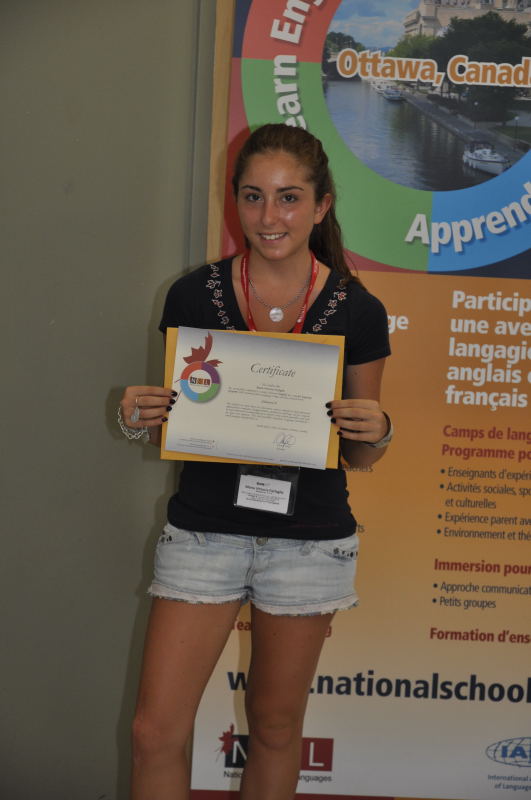This photograph features a young woman, possibly a teenager, with long dark brown hair, pulled back at the top and cascading down her back. She has a tan complexion and could be either white or Latino. Wearing a black v-neck t-shirt adorned with small flowers around the neckline, she accessorizes with various silver jewelry, including a necklace with a round pendant, rings, and bracelets. She is dressed in short, light denim shorts.

The young woman is smiling as she holds a certificate in front of her chest, partially covering a yellow envelope. Her fingernails are painted black. Additionally, she has a red lanyard around her neck with a name tag or ID badge hanging beneath the certificate.

Behind her, there's a colorful poster on the wall that features a circular image of a cityscape with a river, labeled "Ottawa, Canada" in orange letters. The poster includes other information in French, and a plain white wall is visible on the left side of the image.